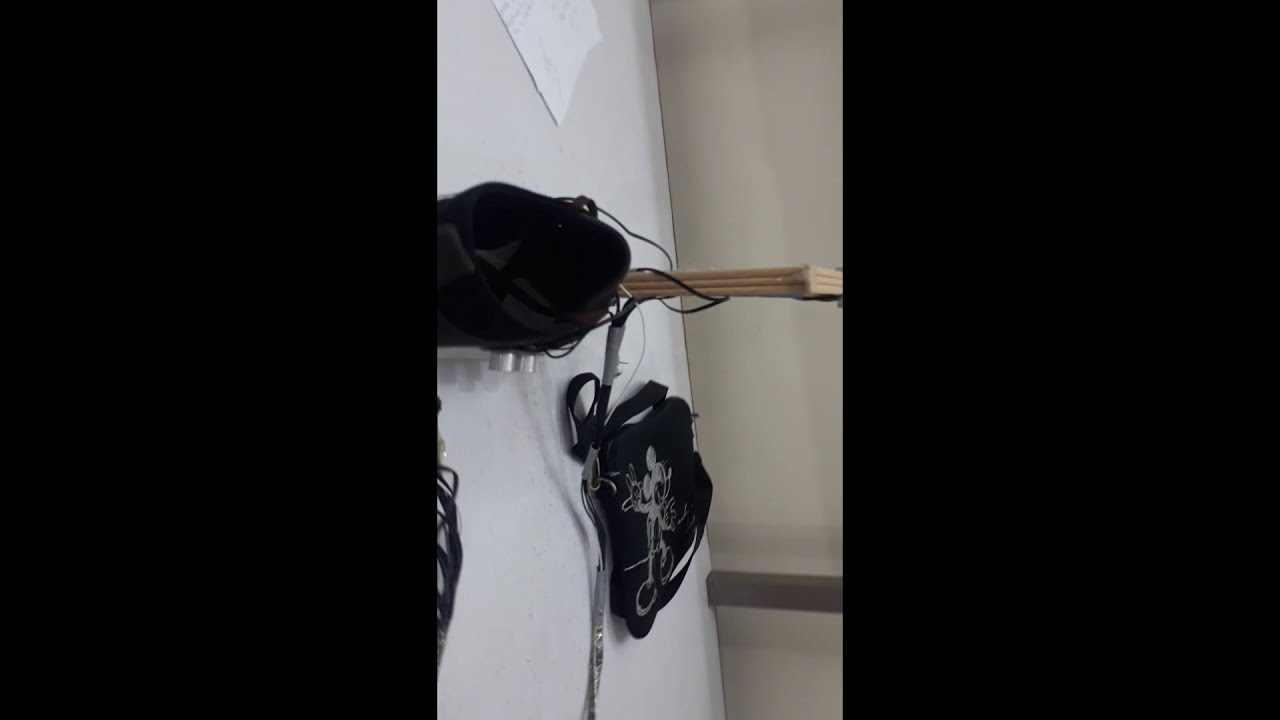The image, shown in a horizontal rectangular format, is divided into three equal sections. The left and right sections are completely black, while the middle section reveals a detailed scene. The main surface appears to be a white countertop, positioned against a beige-tinted wall. On the countertop, there are at least two black bags; one of these bags has a distinctive gray graphic image on it, and the other is located to its left. A white piece of paper lies horizontally on the countertop, situated at the top, which corresponds to the left side of the viewed image. A narrow wooden pole or arm extends from the wall to the countertop, and there are various cords wrapped around this piece. Additionally, there is a metal element protruding from one of the black bags. The scene is bathed in daylight, which illuminates the environment, with light visibly coming from off-frame. Overall, the image presents a mix of materials, including wood, metal, and fabric, arranged in an organized yet somewhat enigmatic manner.